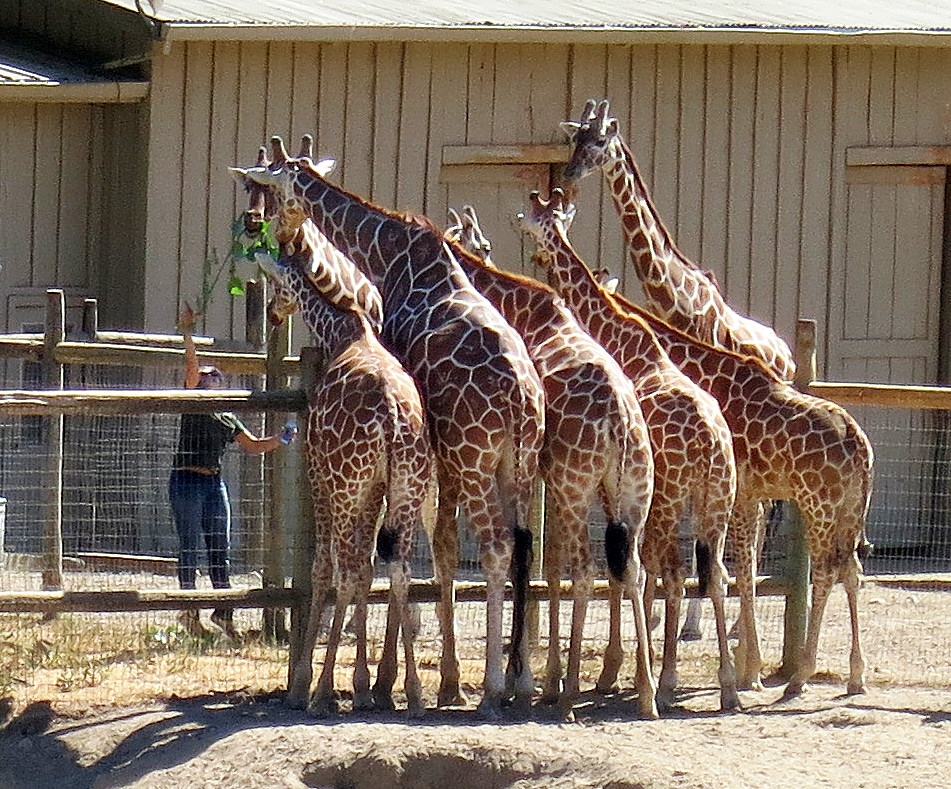In this detailed color photograph taken during the day, six giraffes are gathered at the wire and wooden post fence of a zoo enclosure, eagerly stretching their long necks toward a woman feeding them leafy branches. The ground is a dusty, light brown dirt with sparse patches of grass. The fence, which reaches the tops of the giraffes' torsos, has wooden posts on the top and bottom with wire mesh in between.

The woman, likely a zoo guest rather than a zookeeper, stands on her tiptoes in blue jeans and a short-sleeve black shirt to reach the tall animals. She holds up a branch with green leaves, which two of the giraffes are already nibbling on, while the others wait their turn, forming a semi-circle around her. A wooden shed or barn is visible in the background, and the scene is illuminated by sunlight, capturing a moment of interaction between the visitor and the graceful animals.